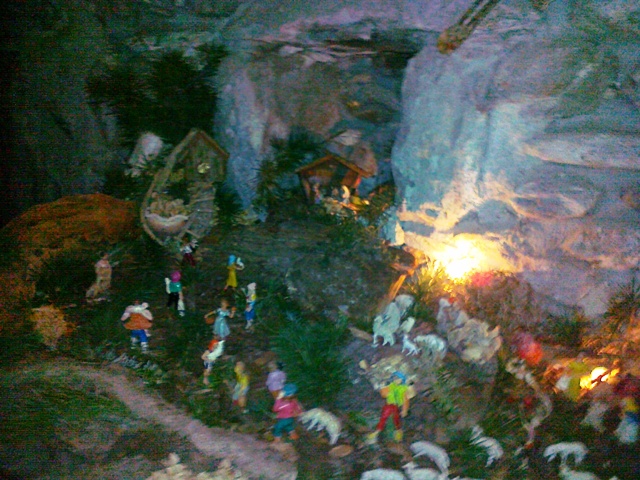The image depicts a distant, slightly blurry scene that resembles either a painting or a photograph of a community or group of figures situated in a lush, green mountainous area. The scene involves small, scattered plastic-like figures, reminiscent of Disneyland or Walt Disney characters, featuring individuals adorned in bright, varied clothing. The figures seem to be part of a lively vignette, possibly incorporating well-known characters like Cinderella, identifiable by her distinctive blue dress. Various animals, particularly white ones, are interspersed among the figures, adding to the intricate tableau. Light illuminates a portion of the rocky mountain terrain—a large cave or hollow on the side of the mountain enhances the ethereal quality of the scene. The image is likely captured from an elevated perspective, looking down upon this vivid, animated slice of life that creates a sense of an enchanted, miniature world.